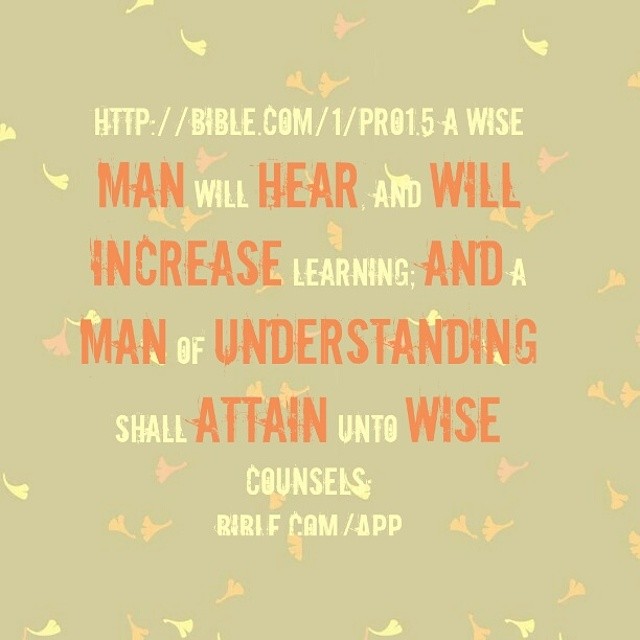This square-shaped image features an inspirational, religious graphic devoid of any headers, footers, or borders. The background is a soft, pale olive color, adorned with subtly falling petals or leaves in shades of yellow, orange, and pink, giving the image a warm and serene feel. Positioned centrally, large bold yellow text starts with a URL: "http://bible.com/one/pro1.5." Below the URL, the quote "A wise man will hear and will increase learning, and a man of understanding shall attain unto wise counsels" is displayed. The key words "man," "hear," "increase," "man," "understanding," "attain," and "wise" are accentuated in a larger, red font, while the remainder of the text is in a smaller, light yellow font. At the bottom, another URL, "bible.com/app," is centered in the same style. This evocative design aims to offer an inspirational and uplifting message suitable for sharing on social media.